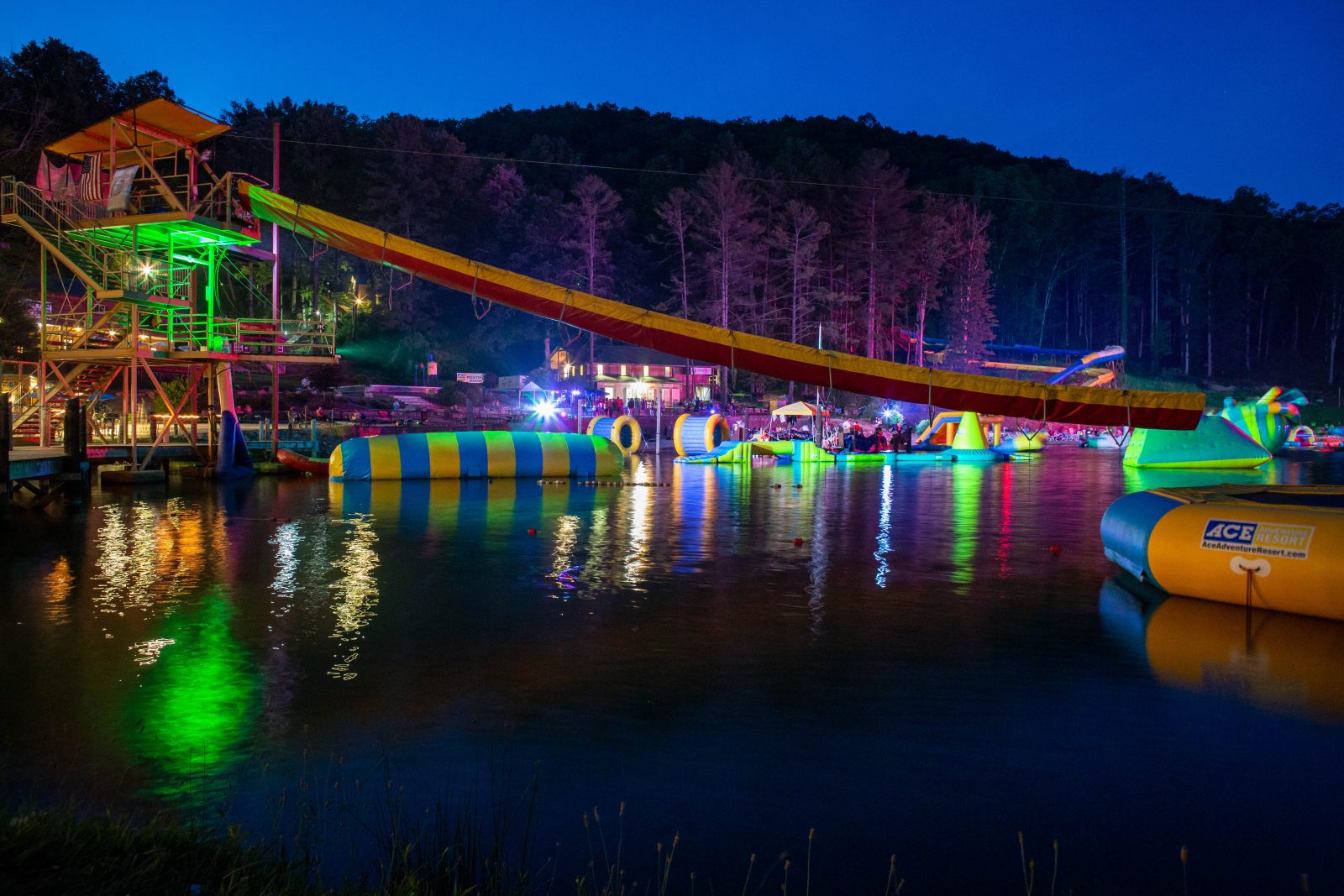This nighttime photograph captures a lively theme park set on a tranquil lake, under a dark blue sky. The distant line of trees frames the background, punctuating the evening scene. The midground features a tower with a green light at its peak, from which a large water slide twists down into the lake, hinting at hours of fun. To the left, a variety of colorful inflatables, including tubes, rafts, and rubber boats in shades of orange, blue, yellow, and neon green, float on the water, adding splashes of color to the dark scene. Reflections of these vibrant colors dance on the lake's surface. Closer to the shoreline, a crowd gathers, illuminated by lights from kiosks and small buildings, possibly a snack bar. The atmosphere is festive and bustling, with people enjoying the nighttime attractions.